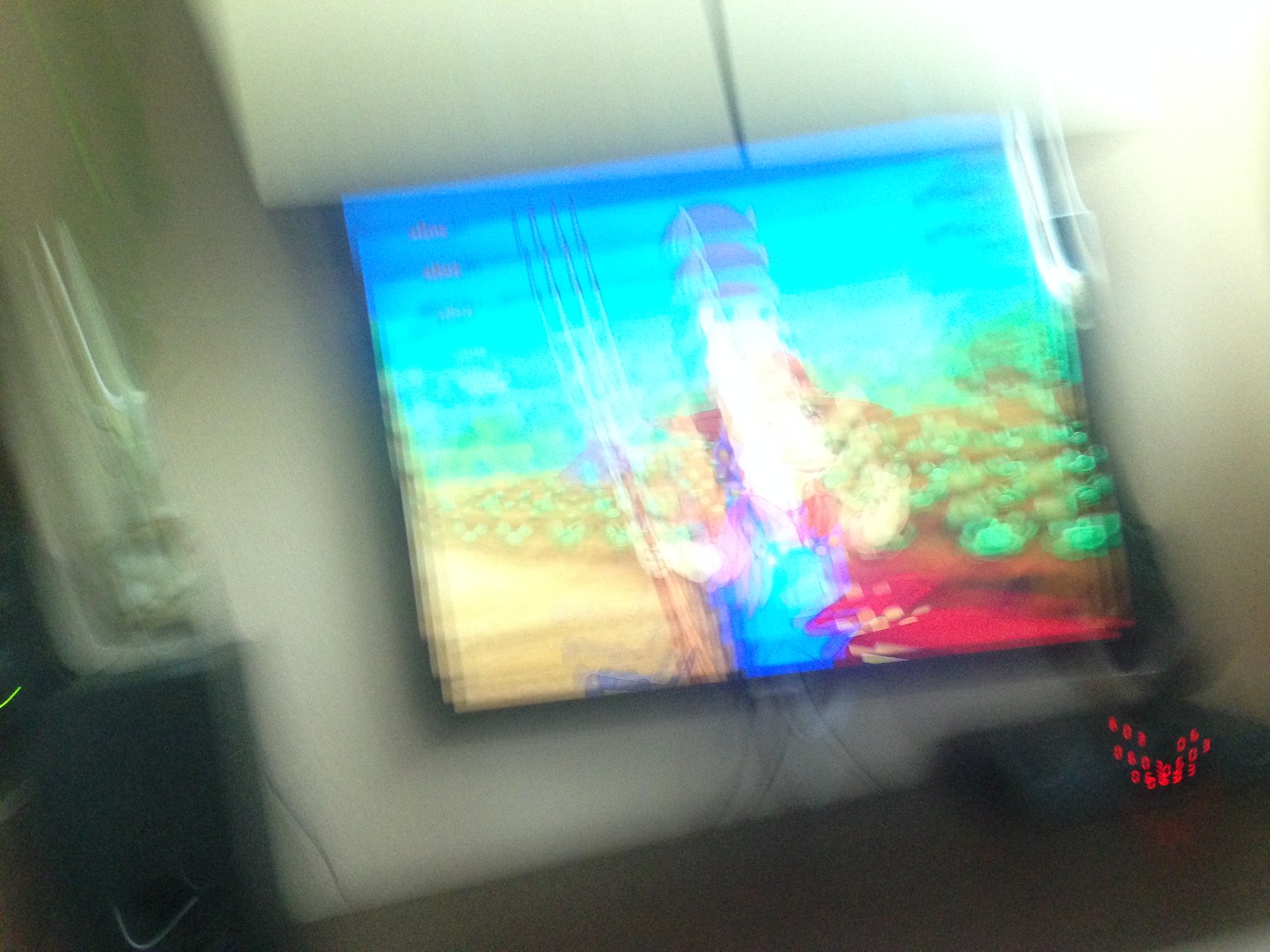The image is a highly blurry shot that appears to have been taken accidentally or with a quick movement, making the details difficult to discern. In the center, there seems to be a tablet screen displaying a colorful cartoon-like image, possibly depicting a farmer tending to a field with a pitchfork in hand. The screen features vibrant hues including light blue, yellow, lime green, red, brown, and white. The tablet is placed on what looks to be a white or leather seat, potentially a chair or a couch, taking up most of the image. Surrounding the tablet, to the left, there's a large, indistinct black piece of furniture, and near the bottom right, there are noticeable red digital numbers or lights, possibly a glowing cord or LEDs. The background features a white neutral-colored wall, with wires hanging down, contributing to the chaotic and indistinct composition of the photo.